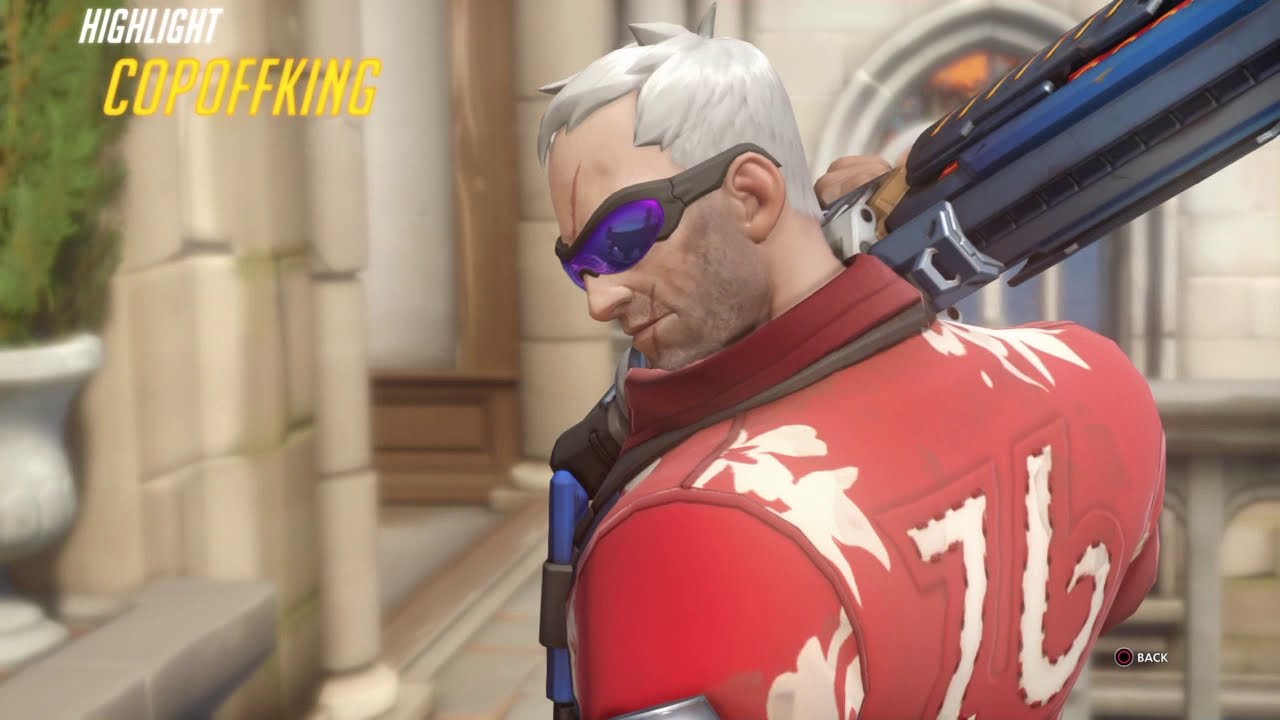The image appears to be a screenshot from a video game featuring a prominently rendered 3D animated character. In the top left corner of the screen, the words "Highlight, Cop Off King" are displayed, with Highlight in white letters and Cop Off King in yellow letters. The character, a man with gray hair and a rough beard, is posing with his back slightly turned towards the camera while glancing over his left shoulder, making his scars—one across his forehead and another extending down past his lips—visible. He is wearing black and purple sunglasses, obscuring his eyes, and a distinctive red jacket adorned with a white floral pattern and marked with the number 76 on the back. In his right hand, which is positioned over his shoulder, he holds a large weapon that features blue, black, and orange colors. The setting around him appears to be the interior of a classic, possibly centuries-old stone building, characterized by large columns and a stained glass window. Additionally, a white flower pot with a tall green plant is situated next to the building, enhancing the historical and serene backdrop.